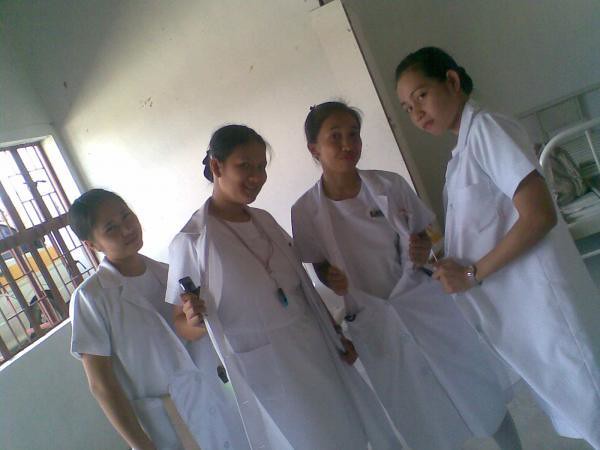The photograph depicts four young women, likely of Filipino nationality, posing together in a hospital setting. Each woman is dressed in a long white coat, which resembles a nurse uniform, complete with white undershirts and lanyards, and they all have their black hair pulled back into ponytails. They are making playful faces at the camera with raised eyebrows and smirking smiles, showcasing a friendly and fun demeanor. The woman on the far right is wearing a watch and making a mock-tough face. The background features a white wall, a bed frame with a glimpse of a white mattress in the bottom right, and a window with a red metal covering on the left. The image quality is poor, but the lively expressions and the clinical setting are prominent.